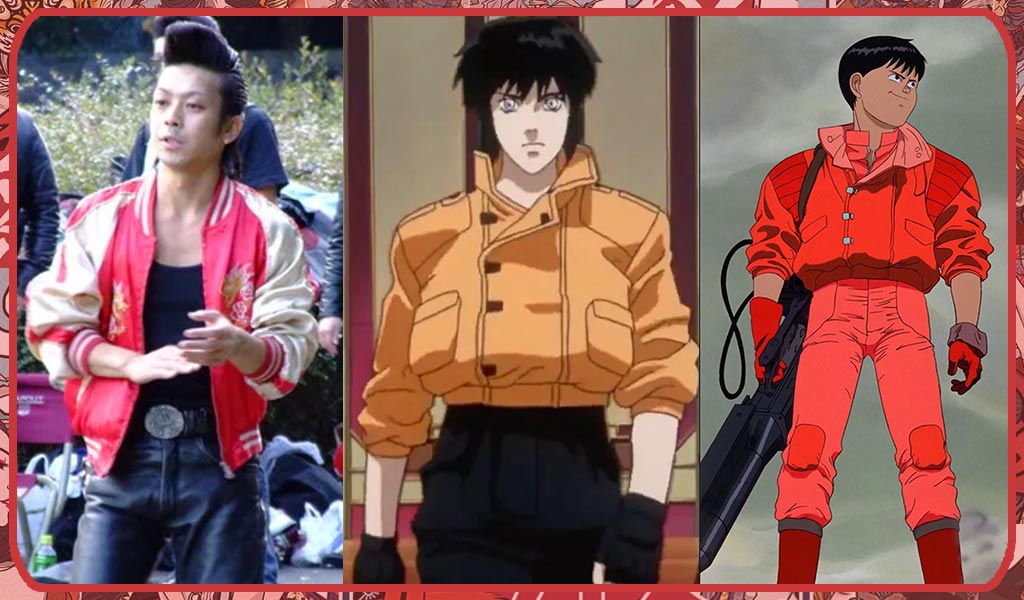This composite image features three side-by-side portraits, combining both photographic and animated elements. The leftmost portrait displays a real-life man of Asian descent, sporting a pompadour hairstyle and dressed in a red and white jacket over a black shirt, coupled with black pants and a large silver belt buckle. He stands outdoors with foliage and other people faintly visible in the background, looking slightly to the left with his hands near his torso.

The central portrait transitions to an animated style, featuring a character with black hair and light blue eyes, clad in a yellow puffer jacket with sleeves rolled to the elbows, black fingerless gloves, and black pants. This character faces the viewer head-on.

The rightmost portrait continues the animated theme, depicting a character with darker brown skin and black hair. He wears a completely orangey-red ensemble, including a puffer jacket, red gloves, and red pants. This character is shown holding a large black object that resembles a weapon, standing against a gray sky backdrop.

All three figures share a cohesive, sleek, and slightly futuristic aesthetic, blending elements of superhero and fighter styles. The entire composition is framed by a vibrant red border and set against a swirling red background, enhancing the unified, dynamic theme of the image.